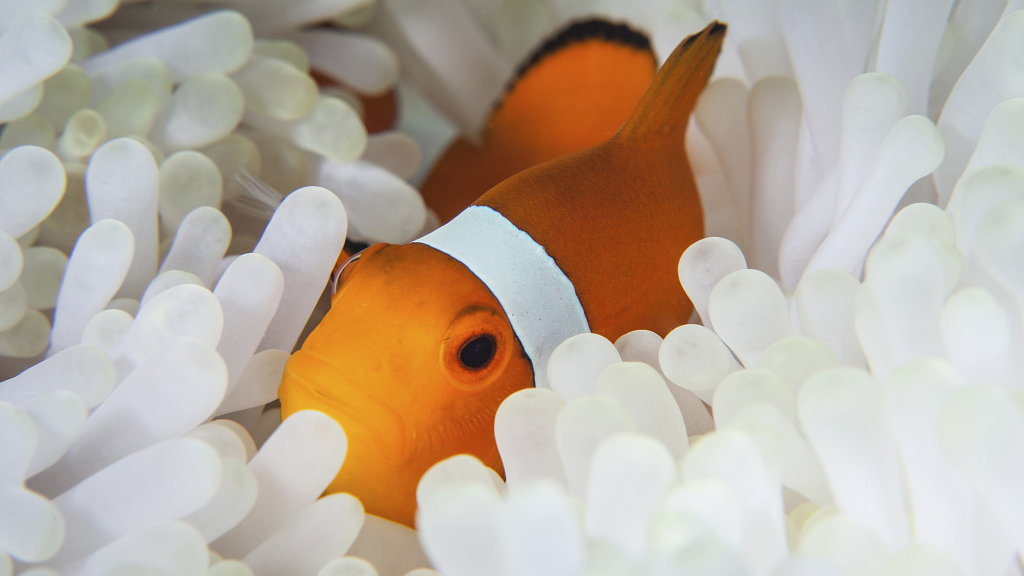The image captures a vibrant scene of a clownfish, characterized by its bright orange face and slightly darker orange body. The fish features a distinctive white stripe bordered by fine black lines, which runs vertically across the center of its body. Its dorsal and caudal fins are accented with touches of black marking. The clownfish is gracefully swimming through a dense cluster of white, tubular sea anemones, which are vividly bright and bulbous. The anemones create an intricate and mesmerizing background, highlighting the clownfish as it navigates through this underwater habitat.